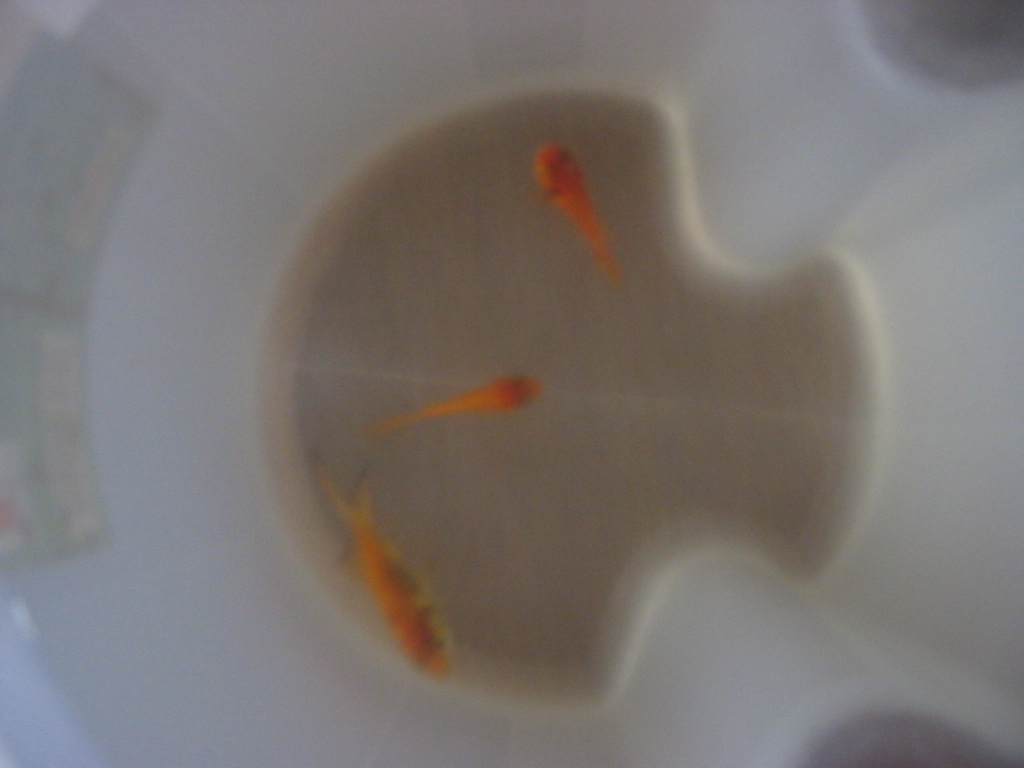The image displays three bright orange goldfish of varying sizes, with one being a bit larger than the other two, swimming in a body of water. The viewpoint appears to be vertical or aerial, making it difficult to discern the exact environment, but there are strong indications that it could be a toilet bowl—evidenced by a thick, white, circular ring resembling a toilet seat surrounding the scene. The background is predominantly white, with a distinctive pattern resembling a tilted mushroom cloud visible at the bottom right side of the image. Despite the blurriness, the fish do not appear lifeless, as they are not belly up and are swimming in different directions without interacting with each other.